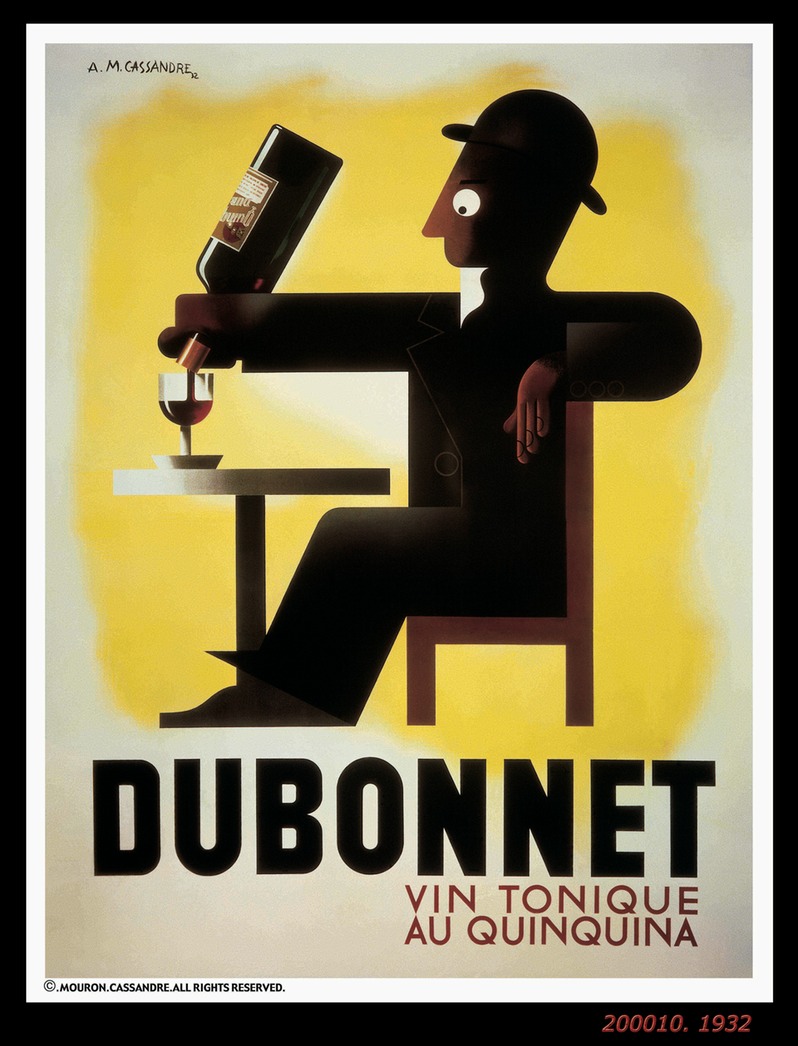This graphic artwork, possibly a poster, is a signed piece by A.M. Cassandre, dated 1932, and includes copyright details "© Mouron Cassandre All Rights Reserved" in the lower left-hand corner. The main image shows a cartoonish profile of a man with brown skin, a black hat, a small white beard, and a straight nose. His face is mostly in shadow, with only his nose and chin visible. The man is seated in a brown wooden chair, his left arm draped over the back, and his right arm extended forward pouring dark maroon wine into a glass on a stone table. The background features a blend of grays and browns, transitioning into a yellow blotchy area in the upper two-thirds. There is also text in the upper left-hand corner reading "Dubonnet Vintonique Quinquina," and a thin black border runs along the outside, followed by a thin white border inside it, completing the detailed and stylized composition.